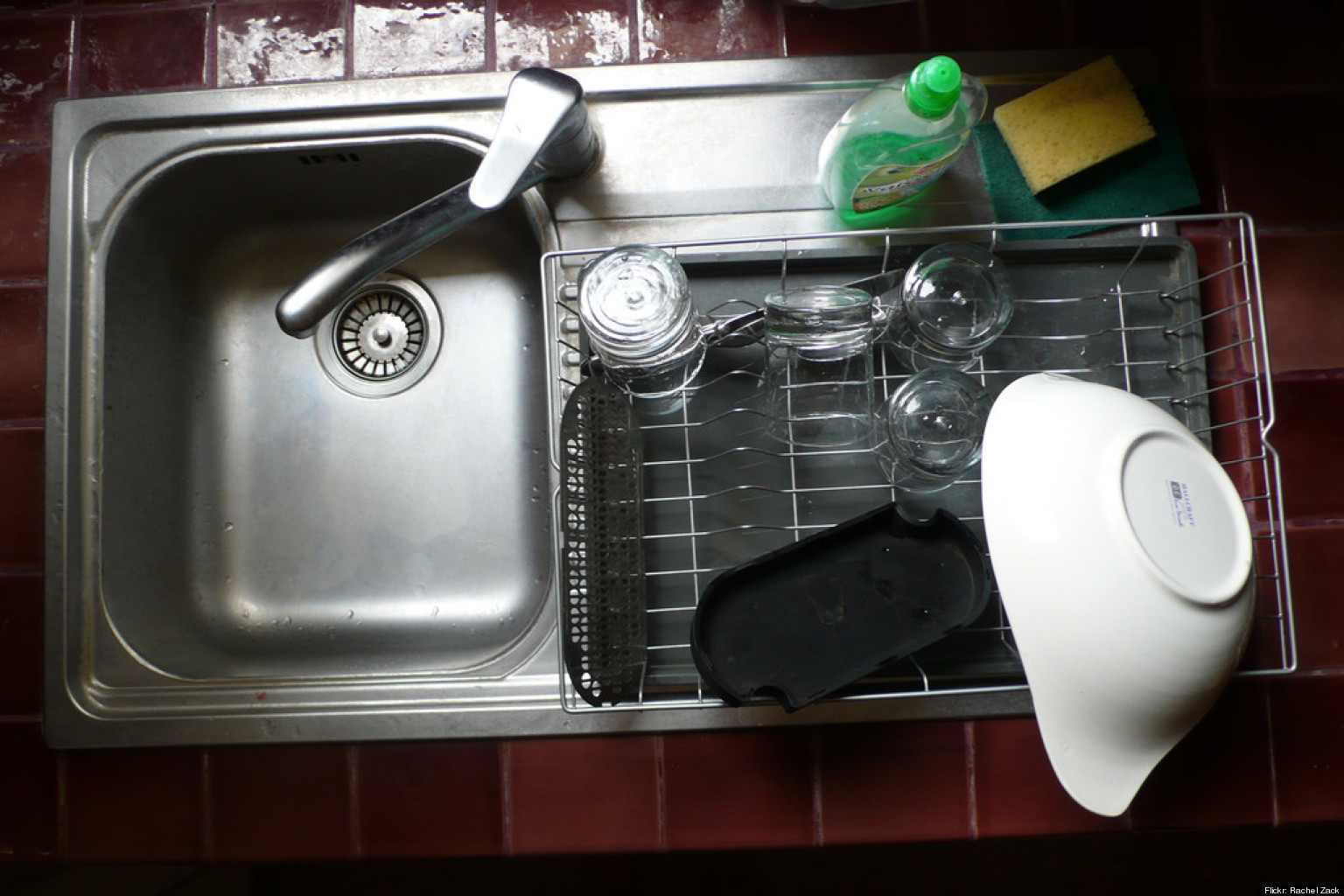A bird's eye view of a kitchen sink and dish rack. The sink, made of silver metal, is split into two sections with the actual sink bowl on the left, where the faucet and single handle spout are located. Surrounding the sink are vivid red tiles. To the right, a metal dish rack holds a white bowl designed for gravy or dipping sauces, four glass cups, a bottle of green dishwashing liquid, and a yellow sponge. At the bottom of the dish rack lies a black plate that appears to be a cup holder. Bright sunlight, likely streaming through a window positioned above or in front of the sink, illuminates the scene. At the bottom right corner of the image, the watermark "Flickr Rachel Zach" is visible.